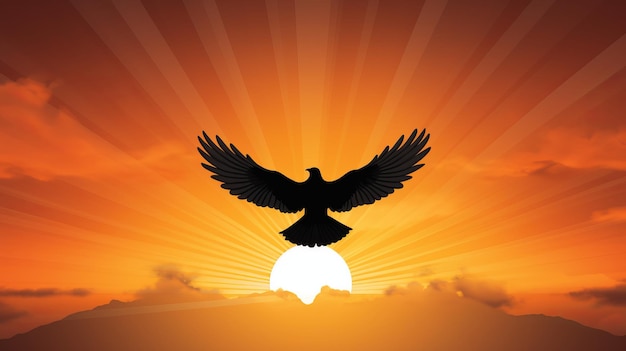The image resembles a striking painting with a vivid orange and reddish-orange background that dominates the entire scene, blending seamlessly into the sky and the ground. The centerpiece is a luminous, neon yellow sun, positioned in the middle at the bottom, either setting or rising, casting beautiful rays of light that scatter across the sky. These rays create a gradient that transitions from bright yellow near the sun to darker shades of orange and brown toward the edges. 

Hovering majestically in the foreground is the silhouette of a large bird, likely an eagle, facing directly forward. The bird appears almost shadow-like, with its wings fully spread out, revealing detailed white tips on its feathers. The eagle’s tail points downward, enhancing its graceful posture as it floats in the air. Surrounding the sun are scattered clouds, adding depth and texture to the orange sky. The entire composition evokes a sense of inspiration and awe, capturing the beauty of nature in a wonderfully abstract and artistic manner.